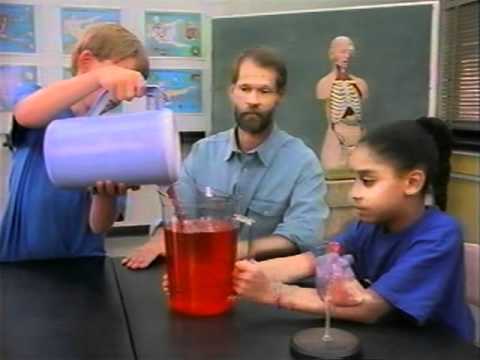The color photograph, likely older and of poor quality, captures a scene that resembles a science class or instructional video. At a black table, a bearded adult male with short brown hair, wearing a blue button-up shirt, sits at the corner with both hands flat on the tabletop, observing two children. To his left, a white boy, about nine years old, stands pouring a red liquid from a large blue pitcher into a clear pitcher. The clear pitcher is being held steadily by a dark-skinned girl, also around nine, who is seated to the man's right in a blue short-sleeved t-shirt. The girl is turned sideways, facing the boy, and supports the clear jug with one hand on either side. The background includes a green chalkboard and a detailed anatomical display model, showcasing a torso with removable organs and visible ribs and muscles. Other educational materials, such as a set of six posters arranged in two rows of three, hang on the wall, enhancing the classroom atmosphere. Beside the girl, to her left, is what appears to be an anatomical model of a human heart, emphasizing the scientific context of the image.